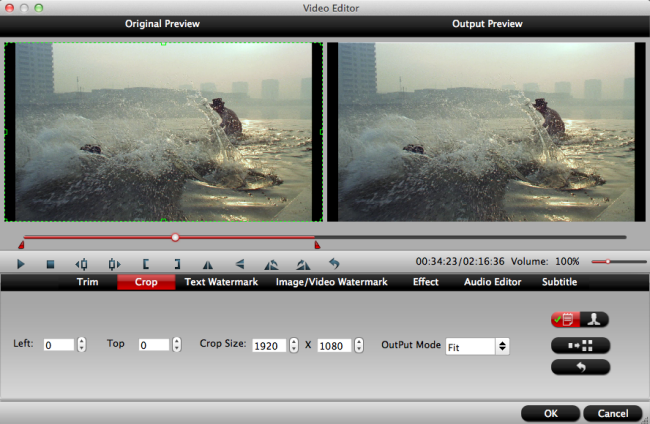This image is a detailed screenshot of video editing software, likely operating on an Apple system, given the signature three dots (red, white, and green) in the upper left corner of the window. Centered at the top, within a gray banner, is the title "Video Editor" written in black text. Just below this, a narrow black bar spans across from left to right. The black bar features two labels in white text: "Original Preview" on the left and "Output Preview" on the right.

Beneath these labels are side-by-side images of a person engaged in a water sport, likely surfing or wakeboarding, with a dynamic city skyline as the backdrop, featuring crashing waves and significant movement. Both images, one under each label, appear almost identical.

Further down, a red horizontal line transitions into a dark gray line from left to right, indicating an editing feature or timeline. Below this line lies another gray panel with various controls and settings, including shapes and numbers primarily in black, and a few in dark gray. A small section features a red box amidst this panel.

At the bottom, another black bar stretches across the width of the window, with white text and controls. The large gray panel below it includes specific editing options such as "Left Top Crop Size Output Mode," accompanied by white boxes containing numerical values. In the lower right-hand corner of this panel are two prominent black oval-shaped buttons labeled "OK" and "Cancel" in white text.